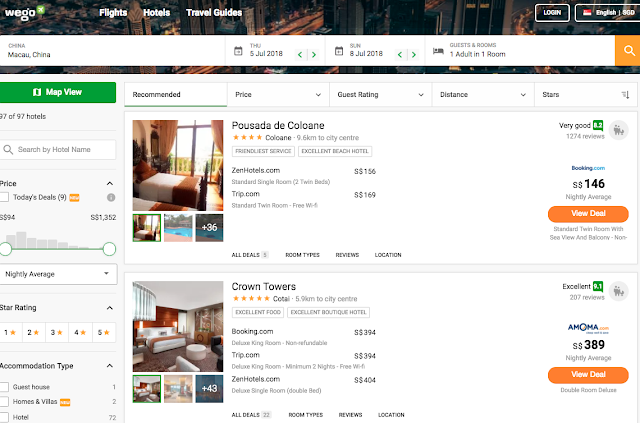Here is a cleaned-up and detailed caption for the described screenshot:

---

This screenshot is from the WeGo (W-E-G-O) website. The top menu bar includes options for "Flights," "Hotels," "Travel Guides," "Log In," language selection (English), and destination details (China, Macau). Date selections are for Thursday, 5 July 2018, to Sunday, 8 July 2018, with one adult in one room specified under "Guests and Rooms." 

On the left-hand vertical menu, users can navigate using options such as "Map View," the total number of hotels available (97 of 97), "Search by hotel name," and filter by "Price" ($594 to $1,352 nightly average). Additional filters include "Star rating" (1 through 5) and "Accommodation type" (Guest House, Homes and Villas, Hotel).

To the right, the sorting options include "Recommended" (underlined), "Price," "Guest Rating," "Distance," and "Stars." 

The photograph displayed showcases a hotel room with two small beds and windows with curtains pulled back, allowing natural light to flood the room. The listing provides details on "Pousada de Coloane" (C-O-L-O-A-N-E), a four-star hotel located in Coloane, 9.6 KM from the city center. The description praises its friendly service and beach location. Booking options are shown from various providers:
- Zenhotels.com offers a standard single room with two twin beds at S$156.
- Trip.com lists a standard twin room with free Wi-Fi at S$169.
- Booking.com highlights the hotel's overall rating as "Very Good" based on 1,274 reviews and offers a nightly average price of S$146, for a standard twin room with a sea view and balcony.

Below this listing, there's another photo of a luxurious room with a large bed, featuring predominantly white and black furniture. This is the "Crown Towers," a five-star hotel located 5.9 KM from the city center. The highlights include excellent food and boutique-style presentation. Booking options are:
- Booking.com offers a deluxe king room (non-refundable) at S$394.
- Trip.com lists a deluxe king room (minimum two nights) with free Wi-Fi at the same price of S$394.
- Zenhotels.com provides a deluxe single room with a double bed at S$404.
The overall rating is noted as "Excellent" with a 9.1 average out of 207 reviews, and AMOMA lists the nightly average price at S$389 for the double room deluxe option.

---